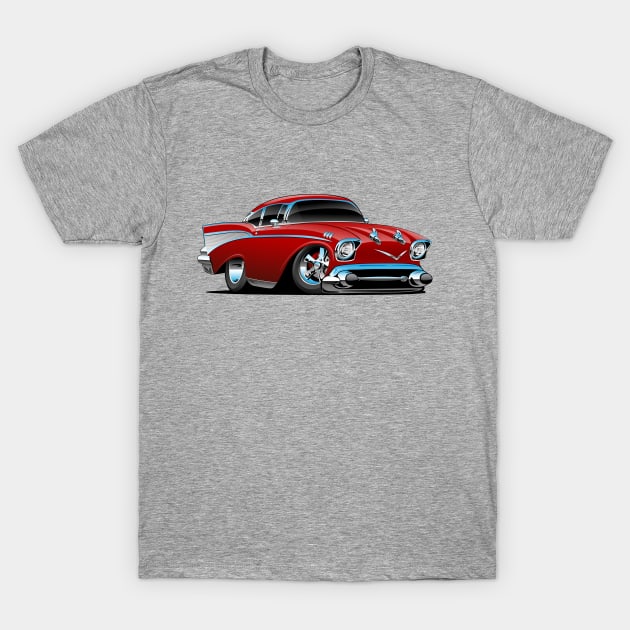This color photograph features a small-sized gray t-shirt, short-sleeved with a crew neck, laid flat against a stark white background. Dominating the center of the t-shirt is an illustrated depiction of a 1957 Chevy, facing to the right. The car is rendered in red with highly exaggerated forms and possesses chrome wheels, a chrome bumper, and other chrome accents that appear almost blue. The vehicle features large round headlights and a prominent grille. A white wing-like design is visible towards the rear of the car, extending down towards the trunk. The windows are entirely black, making them stand out against the detailed body of the car. No tags or text are present on the t-shirt, which is devoid of any extra embellishments.